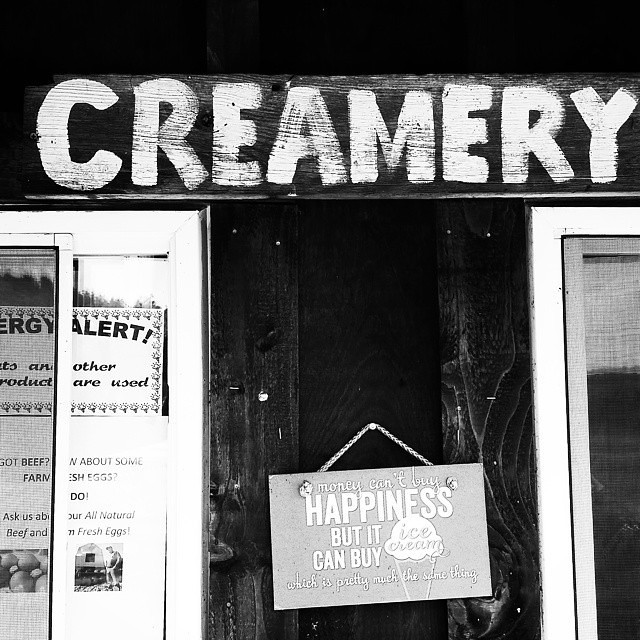This vertical, black and white photograph captures the exterior of a store, prominently featuring a horizontally mounted wooden sign at the top. The signboard, with its clearly visible wood grain, is painted black and bears the word "CREAMERY" in large, white letters. Below the sign is the store's black wood-paneled doorway, with a small decorative item nailed in the center. Hanging from this item, a chain supports a sign that reads, "Money can't buy happiness but it can buy ice cream, which is pretty much the same thing." Flanking the doorway are white-trimmed windows displaying additional signs. One partially obscured sign on the left reads, "Got beef? How about some farm eggs?" and goes on to advertise natural beef and fresh eggs, suggesting the store's connection to local, farm-fresh products.